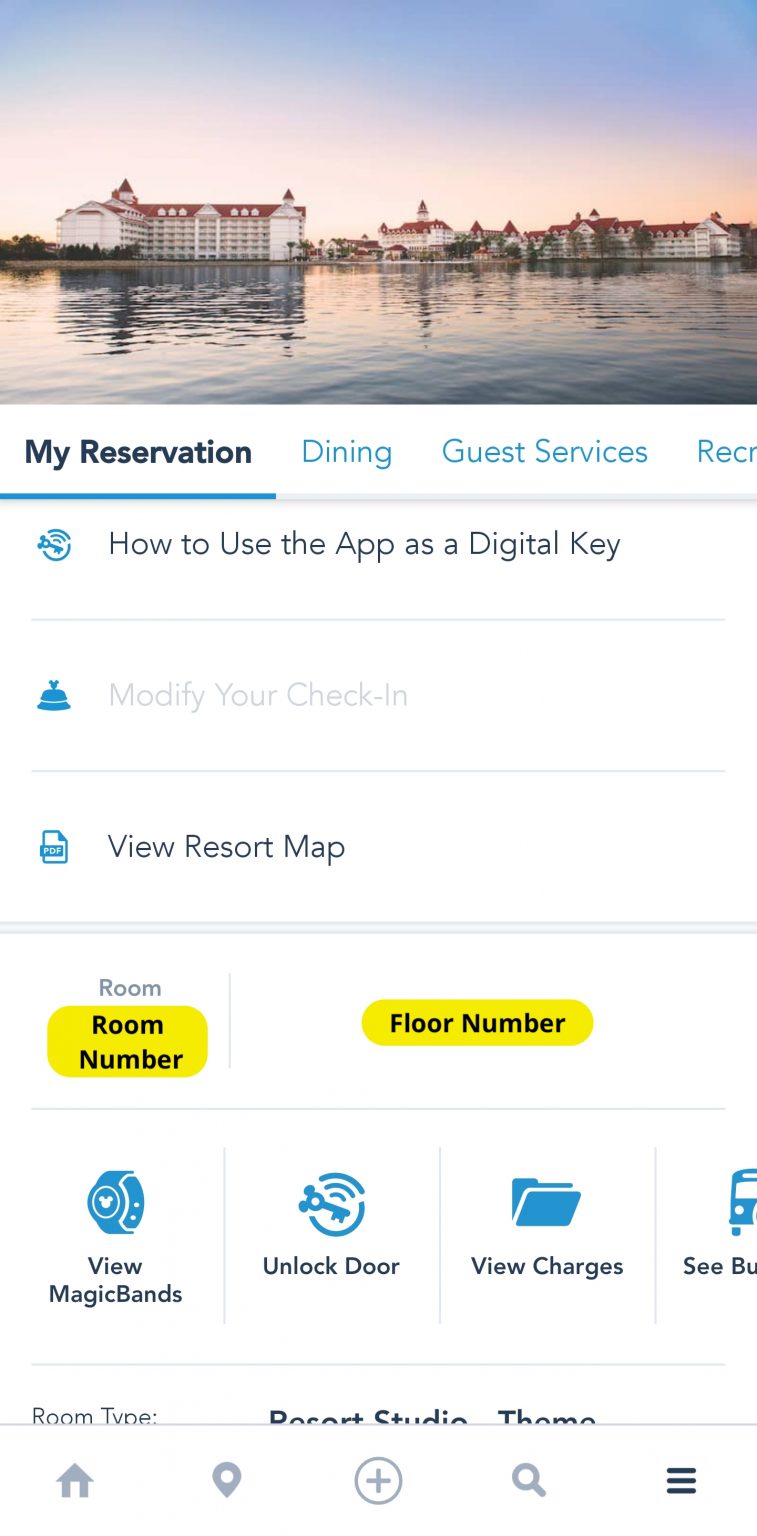The image depicts a "My Reservation" page from a hotel reservation app. At the top of the image, there is a picture of a hotel situated on a waterfront. The foreground of the picture shows a serene body of water leading the eye towards the hotel, which features a distinctive red roof and seems to span multiple floors. The hotel appears to be composed of two sections: a prominent building in the foreground and a larger building in the background, both sharing a similar architectural design.

Below this image, the "My Reservation" tab is prominently displayed, highlighted with black font and underscored by a thin blue line, indicating it is the selected tab. Adjacent to it are tabs labeled "Dining" and "Guest Services".

Further down the screen, there are several interactive options such as:
- Instructions on how to use the app as a digital key.
- A button to view "Magic Bands."
- An "Unlock Door" button.
- A "View Charges" button. 

These interactive elements are neatly arranged, enhancing the user experience by providing quick access to key functionalities of the hotel's app.